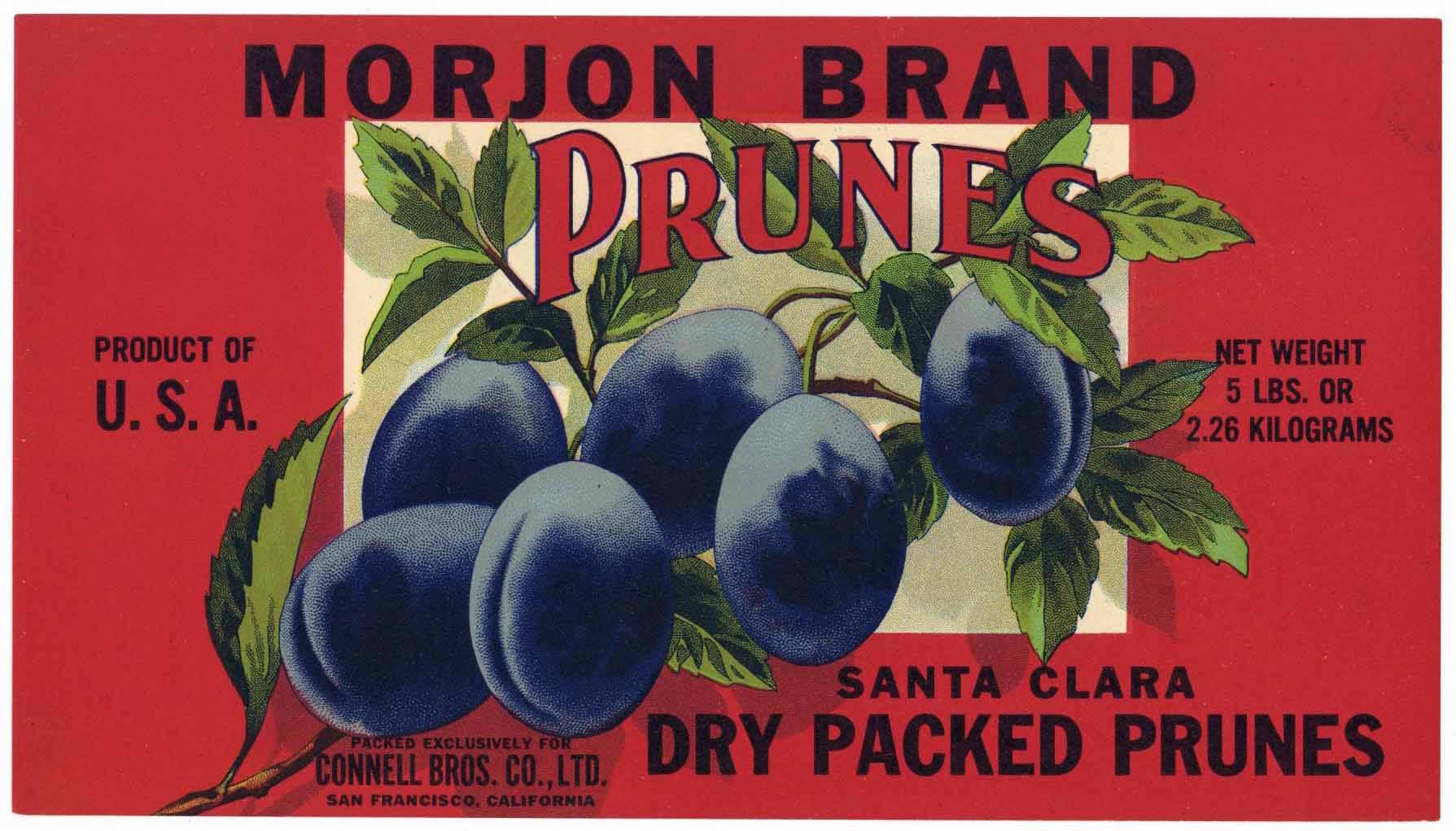This advertisement features a rectangular label with a vibrant red background, predominantly longer horizontally than vertically. At the top, the label displays the text "Morjon Brand" in black capital letters. Below that, there is a prominent white rectangular area with the word "Prunes" written in striking red text. Centrally positioned on the label are six large, dark bluish-purple prunes clustered together, interspersed with green leaves, some arranged in groups of three.

On the left side, in black capital letters, it states "Product of USA." On the right side, also in black capital letters, it mentions "Net Weight, 5 pounds or 2.26 kilograms." 

At the bottom right, in black, larger text, it reads "Santa Clara Dry Packed Prunes." On the bottom left, in smaller black text, it says "Packed exclusively for Connell Brothers Company, LTD, San Francisco, California." The detailed illustration of the prunes and leaves captures a vivid and appealing visual, emphasizing the product's natural and fresh qualities.